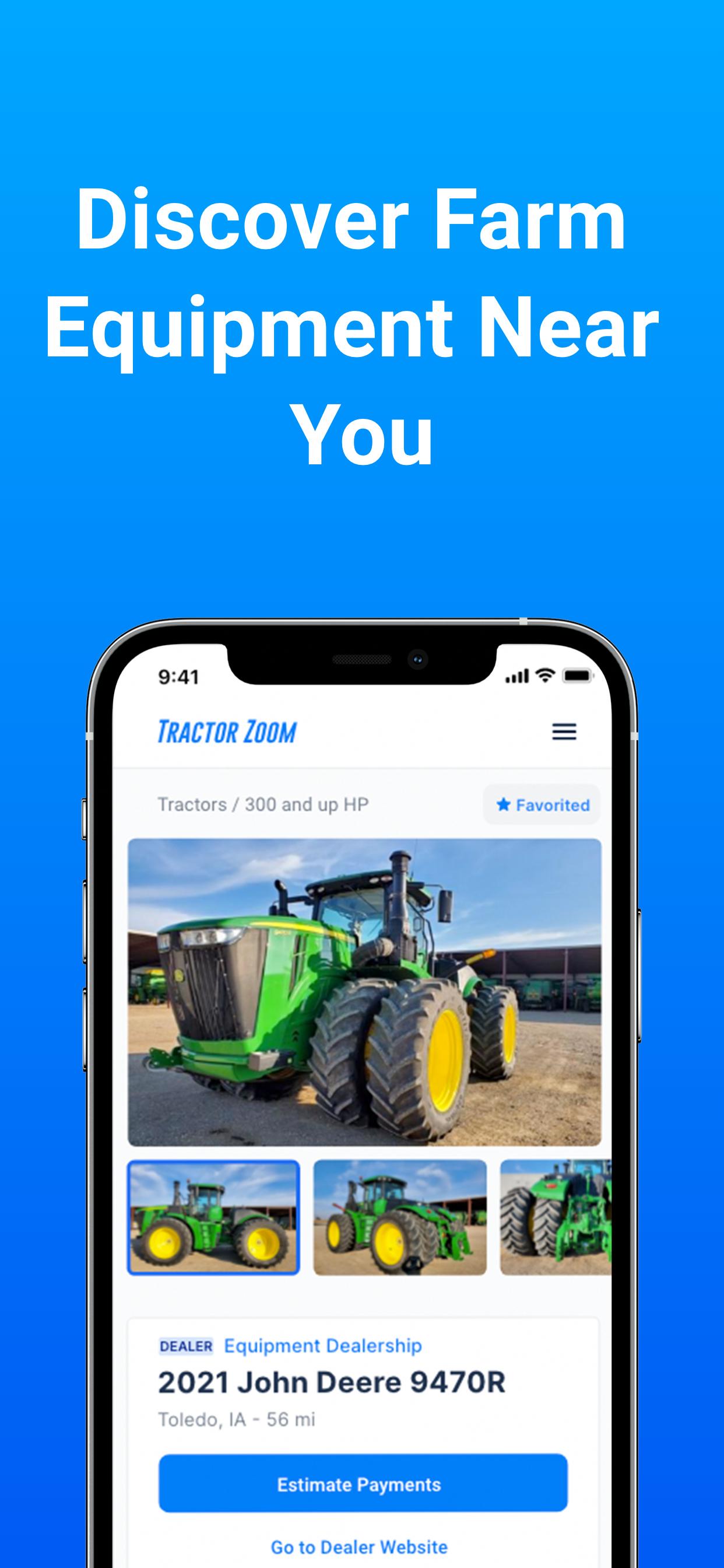**Discover Farm Equipment Near You!**

This advertisement features a large rectangular box with bold white letters at the top that declare, “Discover Farm Equipment Near You.” Below this headline, a smartphone display showcases the Tractor Zoom application. At the top of the phone's screen, it reads "941," with visible connection, Wi-Fi, and battery indicators. The app interface prominently displays "Tractor Zoom" in blue letters on the same line as a drop-down menu bar. 

The next line reads "Tractors / 300 and up HP," adjacent to a blue "Favorited" button marked with a star. Featured prominently on the phone's screen is a large image of a classic green and yellow John Deere tractor. The tractor displays three visible wheels, a large black grill with headlights, and a rear cabin. Beneath this main image are three smaller pictures showcasing different angles of the tractor.

Further down, the ad provides details: "Dealer: Equipment Dealership," "2021 John Deere 9470R," located in "Toledo, Iowa, 56 miles." There is also a blue box stating "Estimate Payments" followed by "Go to Dealer Website."